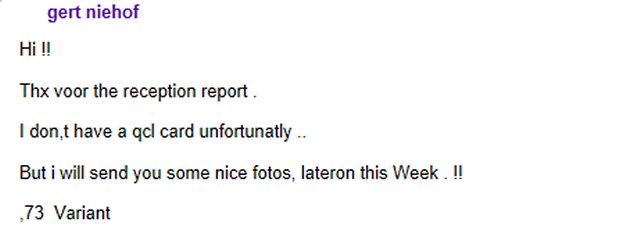The image displays a cropped email or text message with a plain white background and primarily black text. At the top left corner in purple letters, it reads "GERT NIEHOF". Below this, five lines of text are aligned to the left. The first line enthusiastically greets with "Hi!!". The second line abbreviates "thanks" to "THX" and continues, "for the reception report.". The third line states, "I don't have a QCL card unfortunately", where "don't" is mistakenly written with a comma instead of an apostrophe. The fourth line promises, "but I will send you some nice fotos" with "I" not capitalized and "photos" spelled incorrectly as "fotos". This line also combines "later on" into one word. The final line concludes with "73 variant.", indicating informal radio jargon. The text features multiple grammatical errors and informal language.